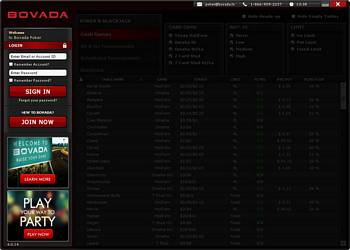The image captures a webpage from the website BOVADA, characterized by its prominent red font. On the left side of the screen, there's a navigation bar featuring options to "Log In," "Sign In," and "Join Now." The central portion of the screen showcases two distinct images. The first image contains the text "Welcome to Bovada," accompanied by a "Learn More" message beneath it, presented as if on a sign. The second image displays the phrase "Play Your World Party" with a call-to-action button reading "Play Now." The rest of the screen is predominantly black with various white fonts, though the text is notably blurry and difficult to decipher. Finally, in the top right corner, there is a prominent red rectangular box with an 'X' symbol for exiting.